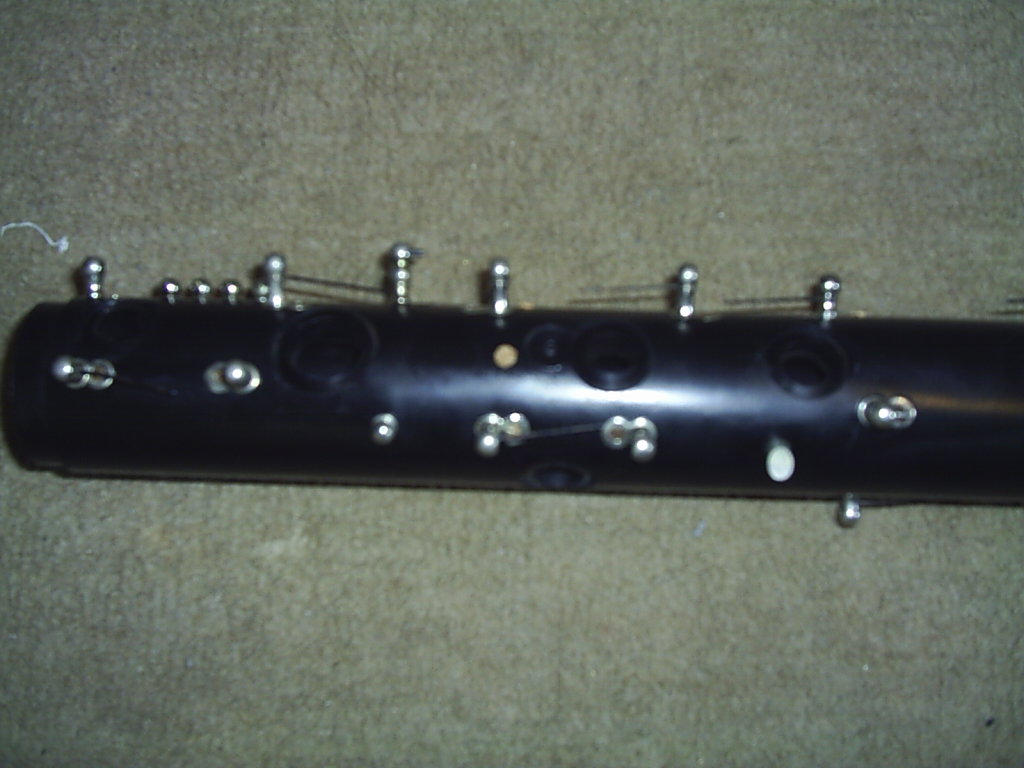The image features a closely taken, slightly blurry photograph of a black cylindrical object, likely metallic, due to the way it reflects light from above. The background appears to be either gray fabric or a clean, short tan-colored carpet. The cylindrical object exhibits numerous small metal pieces protruding from one side, varying in size and appearance. There are around seven or eight metal items evenly spaced or nearly touching in different areas, ranging from a quarter of an inch to fractions of an inch in size. These metal pieces might be pegs, some of which have strings or wire attached, adding to the intricate detail. Scattered along the surface of the object are larger holes, roughly the size of thumbtacks. The object's design, featuring both deeper black grooves and round-topped metal spikes, suggests a possible function, although its specific purpose remains unclear.